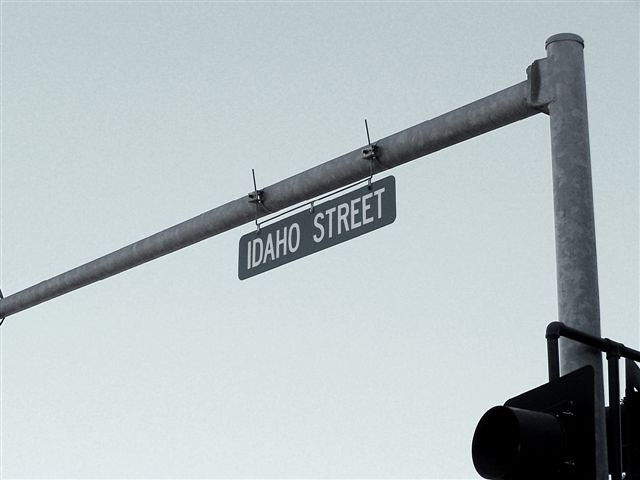The photograph captures an outdoor urban scene under a clear yet grayish sky, which transitions from a darker shade at the top to a lighter hue at the horizon. Central to the image is a steel signpost, vertically extending upwards before jutting out horizontally. At the top of the post hangs a street sign, prominently displaying "IDAHO STREET" in capital white letters against a dark gray background. Supporting the sign, metal chains securely fasten it to the post. To the right of the signpost, partially visible within the frame, is a traffic light, specifically the top section designated for the red signal, though the light itself remains unseen due to the angle of the photo. This traffic light is affixed to the signpost through a sturdy metal grate, contributing to the structure's overall industrial aesthetic.